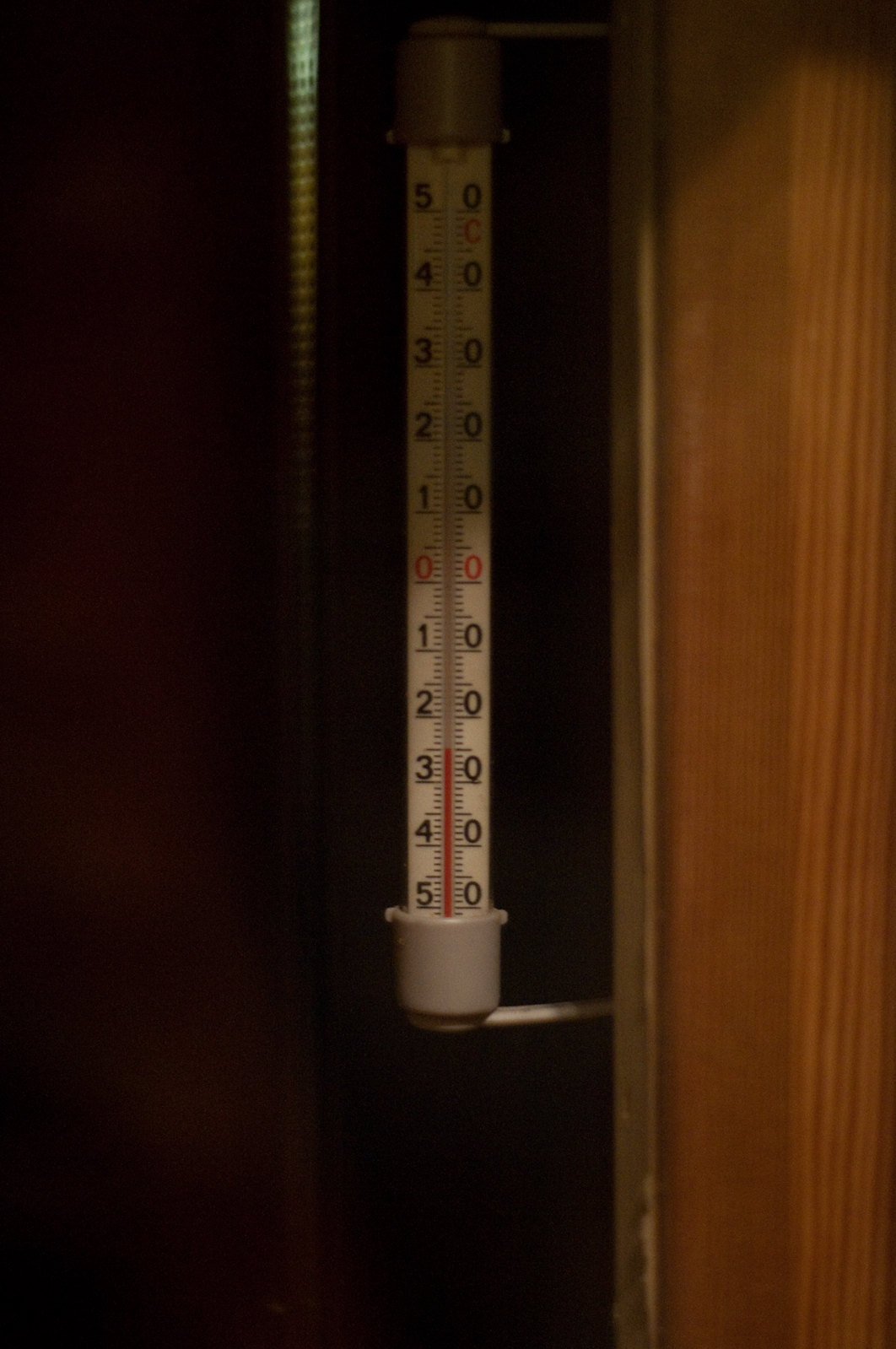The image features a close-up view of a thermometer mounted on a wooden wall. Despite the slightly shaded setting, the items in the image are clearly identifiable. The thermometer, encased in a metal frame, displays temperature readings in degrees Celsius. The scale on the thermometer ranges from -5 to +5 degrees. The red liquid column within the thermometer indicates a current temperature of approximately -2.5 degrees Celsius. The placement of the thermometer on the wooden wall gives it a suspended appearance, as it is installed at a noticeable height.